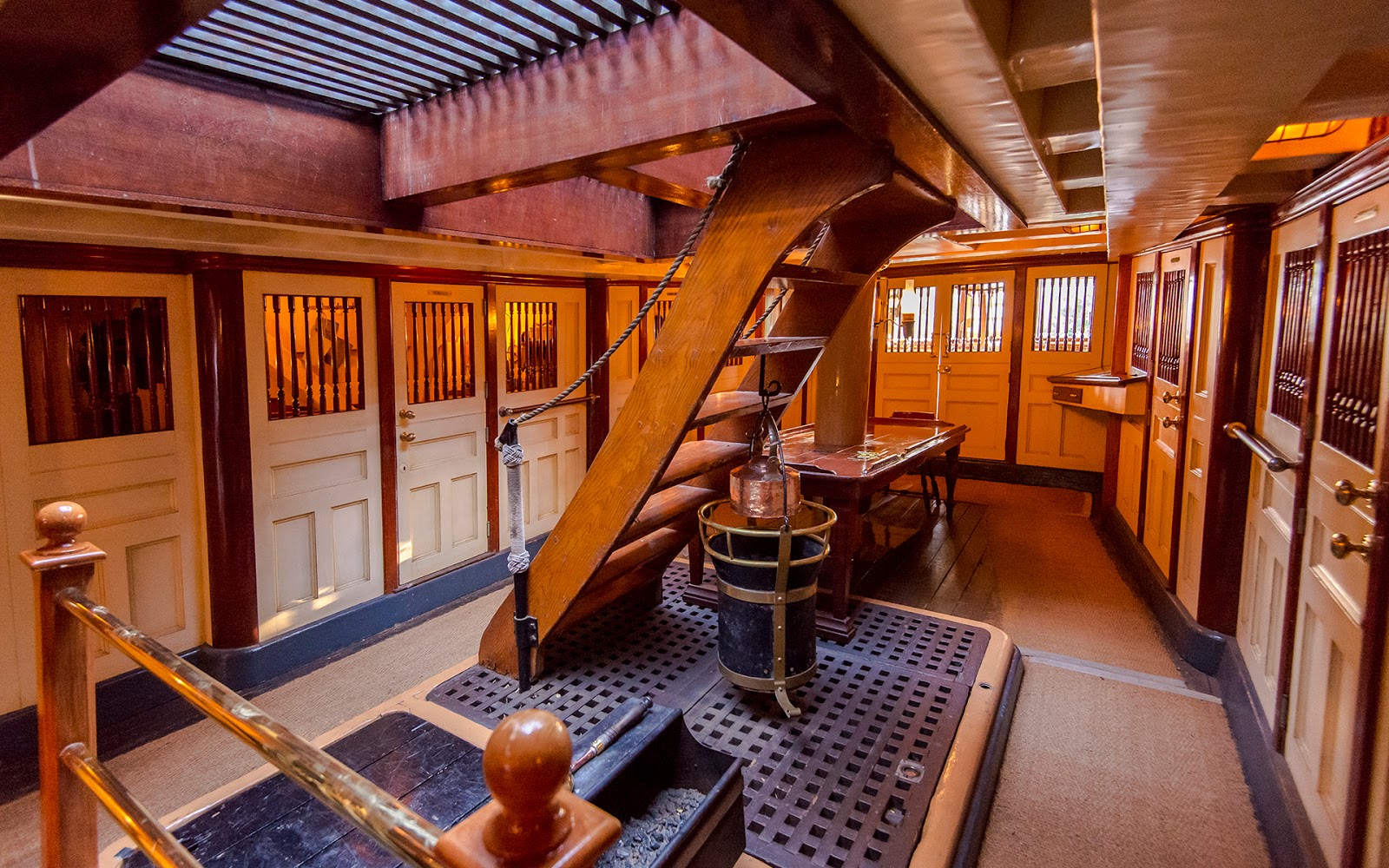This photograph captures the inside cabin of an antique wooden ship, revealing a detailed glimpse into its close quarters. Centered in the image is a narrow wooden staircase descending from the top deck, flanked by rope handrails and leading into the densely packed cabin. The cabin is enveloped in a rich, wooden frame with wooden doors closely positioned along the left side, suggesting tight quarters akin to old nautical designs. Light filters generously through a ventilated metal grate overhead, which also allows sunlight to spill into the otherwise dim space. To the right of the staircase lies a table with an aged chair, emphasizing the rustic, preserved nature of the setting. Opposite the staircase, within the cramped room, are multiple white doors, possibly leading to small compartments or closets, each equipped with antique doorknobs and wooden railings resembling jail cells. The room features a beige carpet, and a small desk cutout area is tucked into the back, adding a functional touch to the historical layout. Overall, the decor and fixtures emanate an historical, old-timey ship feel, possibly designed for preservation and tourist exploration.